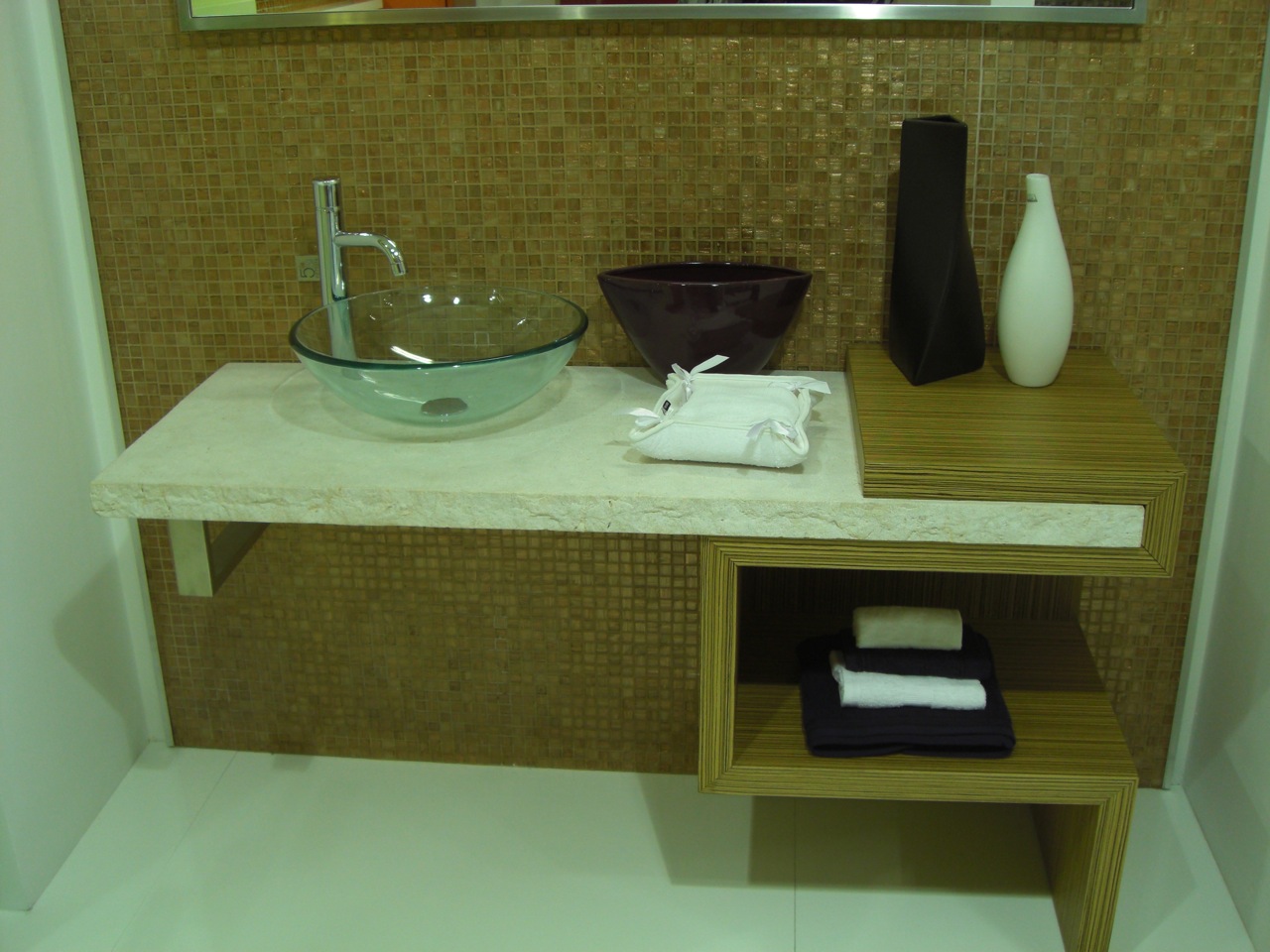The image depicts a modern, minimalist bathroom design with a distinct geometric style. Dominating the scene is a tiled wall composed of tiny square tiles in varying shades of gold, copper, and silver. Built into this wall is a sleek white shelf, on which rests an assortment of decorative items: a transparent round glass bowl located directly beneath a projecting chrome faucet, a square brown open bowl, and several other design artifacts. Below the white shelf, a wooden shelf holds neatly folded towels, showcasing both practicality and elegance. At the top edge of the image, the corner of a mirror is visible, adding depth and reflecting the room's clean lines and contemporary aesthetic.